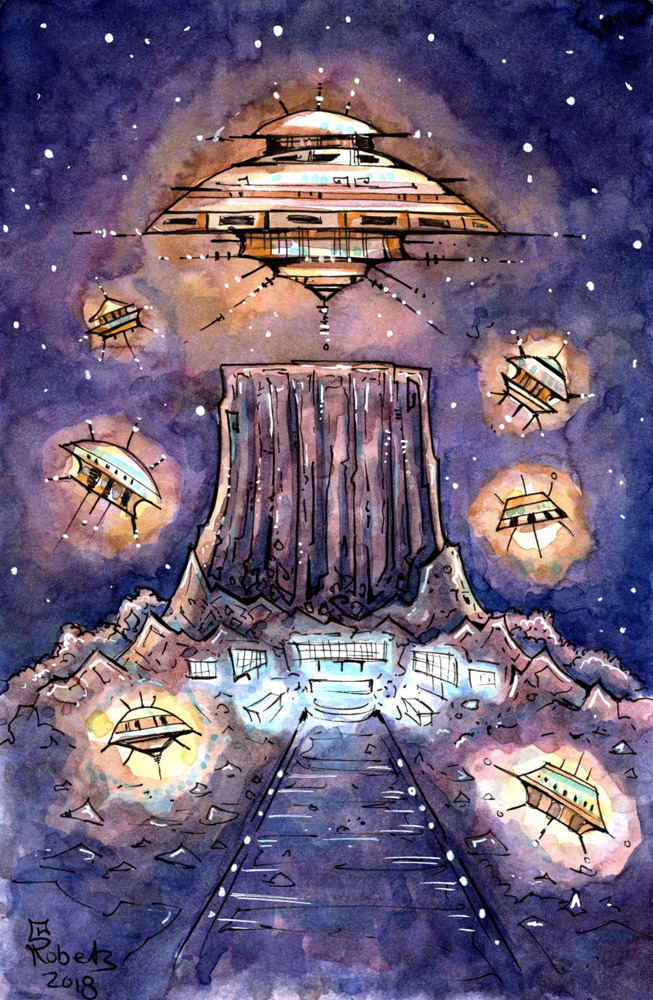The image is a detailed, hand-drawn sketch depicting an alien encounter set against a night sky. The primarily purple and blue background, dotted with white stars, illustrates a mountainous terrain with a towering peak at the center. Nestled in the foothills of this mountain is a small town, illuminated by blue-lit buildings with square windows. A winding path leads directly to these structures, which are positioned centrally in the composition. Dominating the sky above the town is a large mothership, flanked by six smaller glowing alien ships—three on each side—casting an eerie orange and yellow light. The scene is imbued with a sense of impending science fiction drama, capturing the viewer’s imagination with its vibrant colors and detailed portrayal of a UFO invasion.